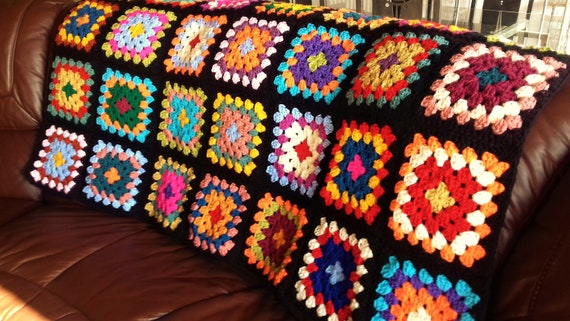The photograph depicts a vibrant knitted quilt draped over the back of an auburn brown leather sofa. The quilt features a black background accentuated by an array of brightly colored squares, each with intricate multi-layered patterns. Visible are seven squares wide, across three rows, with more partially folded over the back of the sofa. These squares showcase a kaleidoscope of colors including white, red, light blue, yellow, turquoise, purple, orange, hot pink, maroon, and various shades of green. Each square comprises four distinct levels of design, with the outermost layer often adorned with tiny oval or ball-shaped motifs, followed by zigzag patterns, culminating in a vibrant central color. The lower section of the quilt displays a striking white square with successive layers of red, light blue, and yellow towards the center, next to a square with light blue, orange, and dark blue segments. The overall effect is a dynamic, colorful display that contrasts vividly with the brown leather of the sofa.